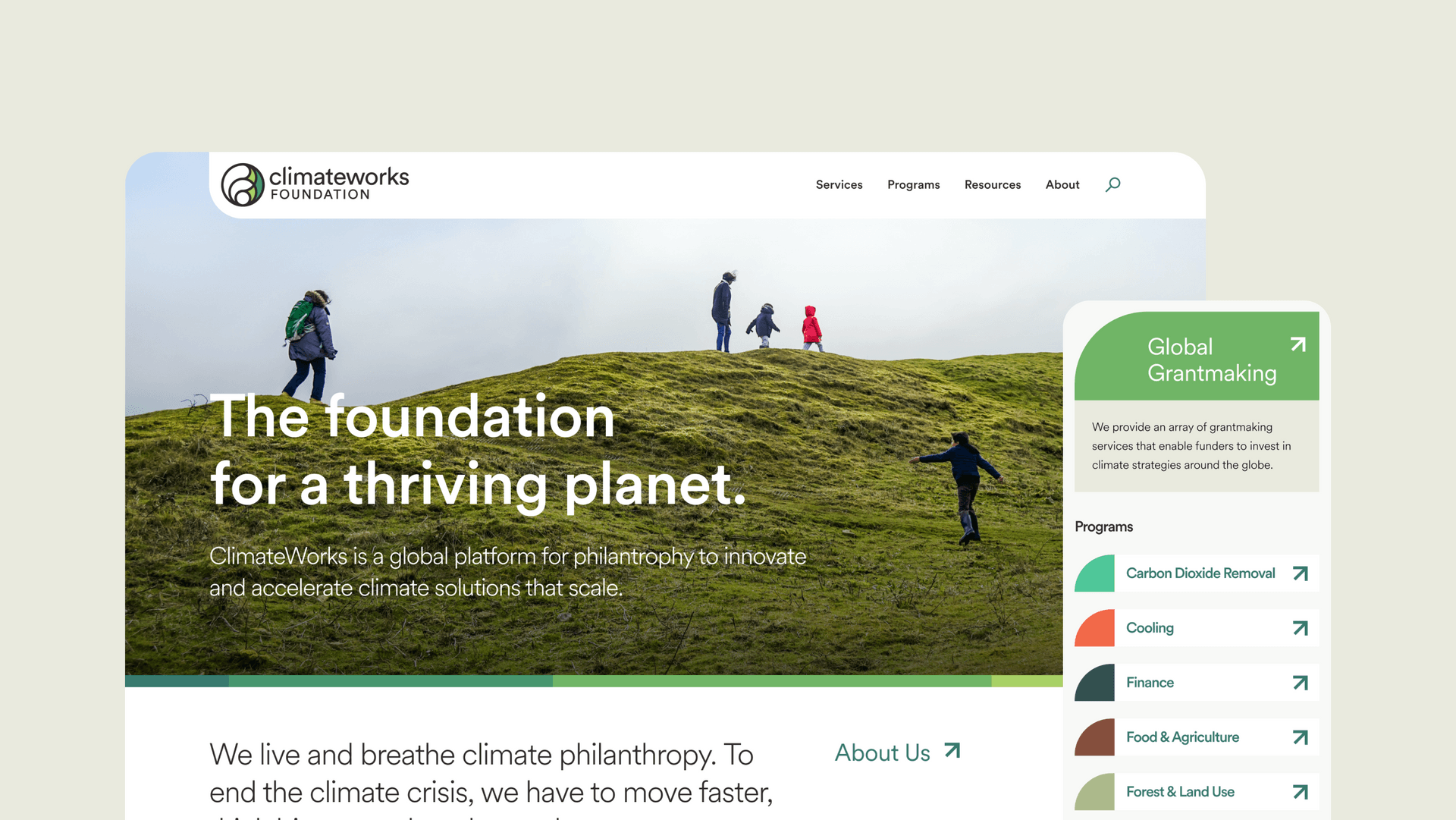The image showcases a partial view of the ClimateWorks Foundation website. On the left, a section is highlighted with the text "Global Grant Making" overlaid on the image. The website's logo, "ClimateWorks Foundation," features prominently at the top, with an accompanying icon of a large circle containing two smaller circles, rendered in a certain color.

To the right of the logo, a navigation bar spans the top of the site, displaying menu options: "Services," "Programs," "Resources," and "About," along with a magnifying glass icon indicating a search function. This navigation bar is set against a white banner that nearly covers the top width of the image.

In the background, a scenic image depicts a mountainous area, with a family of five gazing at the landscape. Overlaid text reads, "The Foundation for a Thriving Planet," followed by a small, two-line sentence.

The image cuts off with a text ending at "we live and breathe climate philanthropy. To end the climate crisis we have to move faster,." On the right-hand side, the word "About Us" appears, with an arrow pointing toward the "Global Grant Making" section.

Below this, a light gray box contains a paragraph, beneath which is a header titled "Programs." Here, several colored icons represent various initiatives: "carbon dioxide removal," "cooling," "finance," "food and agriculture," and "forest and land use." Arrows point diagonally to the right for each listed program.